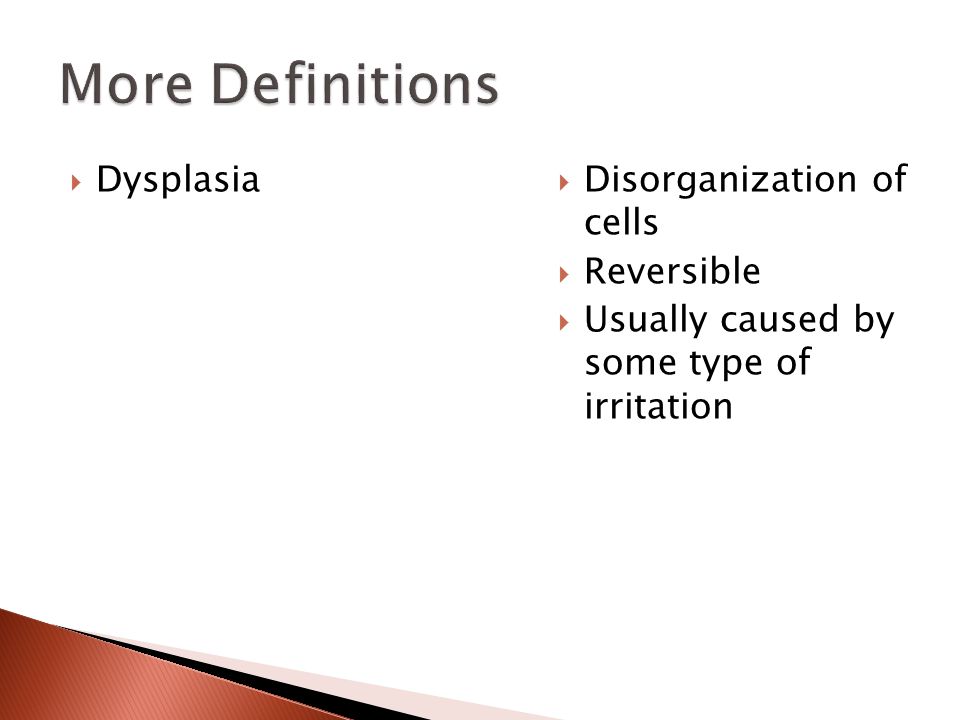The image depicts a screenshot of a PowerPoint slide, with a clean and minimalistic design. The slide has a title at the top left that reads "More Definitions." Below the title, the term "Dysplasia" is prominently displayed. To the right of this term, there is a concise definition: "Disorganization of cells, reversible and usually caused by some type of irritation." The text appears to be the sole content on this slide, designed to provide a clear and straightforward explanation. The design of the slide includes a rust-red colored accent at the bottom left, adding a touch of visual interest and aiding in the overall aesthetic coherence of the presentation.